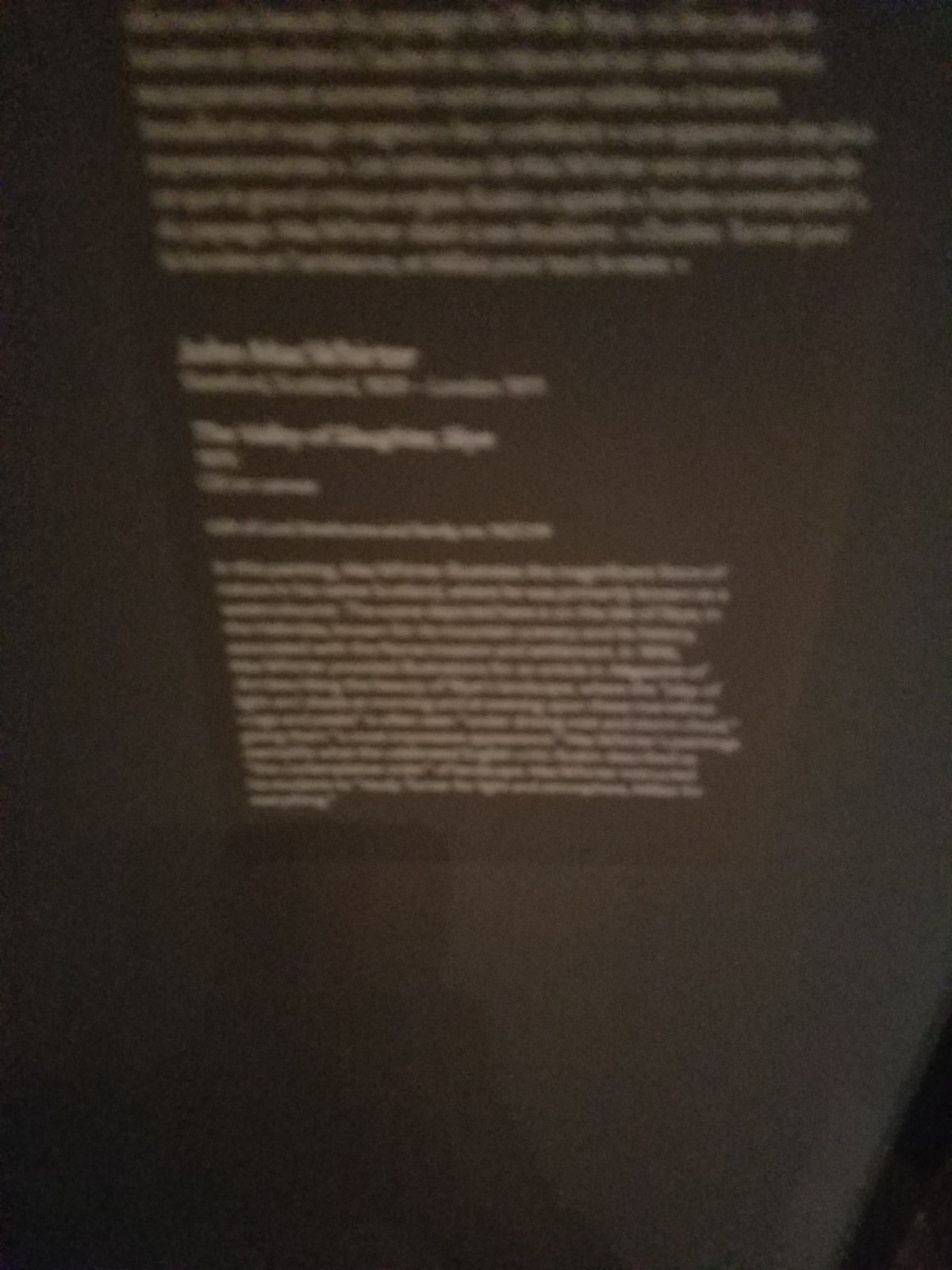This photograph captures a computer monitor displaying a text log. The screen border is deep black, complementing the dark gray background of the display. In the reflection on the monitor, a faint shadowy silhouette of the photographer is visible. Dominating the center of the screen is a rectangular box filled with white text. Although the text is too blurred to discern specific words, the structure suggests it consists of a paragraph, followed by a couple lines of separation, and then another paragraph, forming a cohesive block of information.